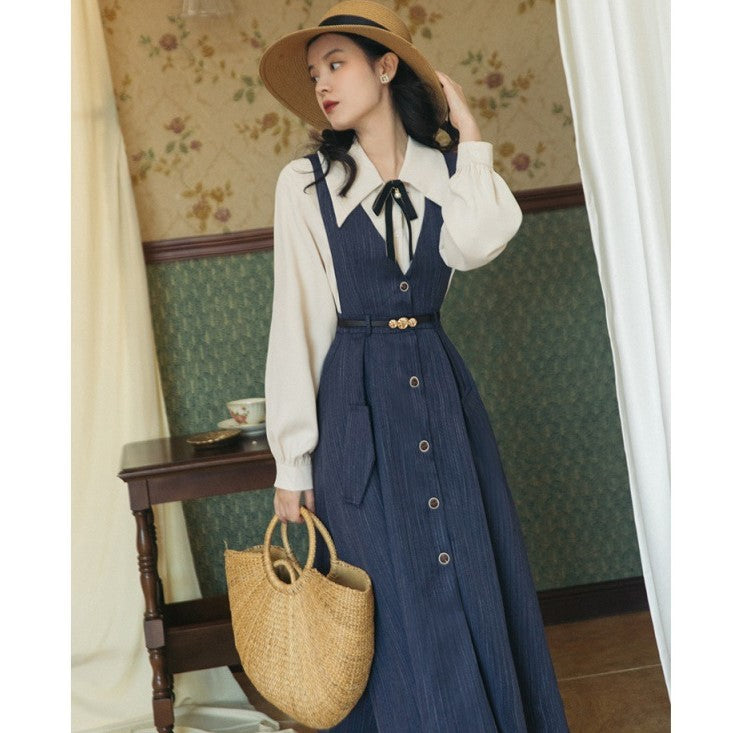A young Asian woman is elegantly posing in a navy blue pinafore dress with a deep V-neck and five metal buttons down the front. The belt at her waist is black, adorned with three brass-colored buttons, with the middle button being larger than the others. She wears a white blouse underneath, featuring very large collars that nearly reach her elbows and puffy sleeves. A black bow is tied at her neck. Her dark black hair falls past her shoulders with some volume, and she has large earrings. She has a broad-brimmed tan straw hat, accented with a black ribbon, positioned stylishly on her head. In her right hand, she holds a woven straw bag, and her left arm is bent at the elbow, hand resting on her hat.

The background is a vintage home setting. There are white curtains that run diagonally, creating an illusion due to the tilted angle of the photograph. The upper part of the wall is adorned with tan wallpaper decorated with red and yellow rose-like flowers surrounded by green leaves, while the lower section features sage green wallpaper with criss-crossing diagonal lines of white patterns. Between these sections, a horizontally stained mahogany wood trim adds a classic touch. In front of the curtains, on the left, there is a low, rectangular wooden table with carved legs, also stained mahogany. Atop it sits a white Victorian-style teacup with red floral patterns and possibly a bronze or gold ashtray or plate. The overall aesthetic suggests this might be a photographed scene from a fashion magazine, capturing a blend of vintage charm and modern elegance.